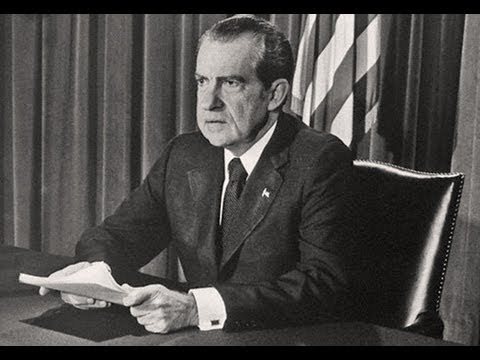This black-and-white photograph captures President Richard M. Nixon seated in a glossy black leather chair at a desk in the Oval Office, circa early 1970s. Nixon is shown in a three-quarter view angle, facing the left, showcasing his stern and concentrated expression as he addresses the public, likely through a television camera. He is dressed in a dark suit complemented by a white button-down shirt, a black tie, and an American flag pin on his left lapel. His dark brown hair, slightly peppered with gray, is combed back. The cuffs of his white shirt and elaborate onyx cuff links peek out from his suit sleeves. Nixon's forearms rest on the black table, casting a shadow, while his hands hold a stack of papers, slightly tilted upward. Behind him, the iconic draped curtains of the Oval Office can be seen, along with a prominent American flag standing just behind his head, framed by some gray wall panels.